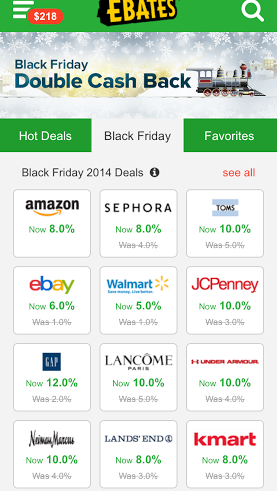The image is a smartphone screenshot featuring the Ebates (now Rakuten) app interface. At the very top, a bright green border frames the screen, drawing attention. Centrally placed is the Ebates logo, prominently displayed in yellow capital letters with a black outline. In the upper right-hand corner, a circular search icon aims downwards to the bottom right, indicating a search function. On the upper left, three horizontal white lines suggest a menu button for accessing other pages. Adjacent to this is a red oblong shape with a white dollar sign followed by "218," presumably indicating the cashback amount.

Beneath this section, a festive graphic with a light gray sky and falling snowflakes sets a seasonal tone. Overlaid on this backdrop, in gray font, the text reads "Black Friday, double cash back." To the right of the word "back," there is a simple illustration of an old-fashioned steam engine train, adding a whimsical touch.

The remainder of the image features tiles with the names and logos of well-known stores. Among these are Amazon, Sephora, Ebay, Walmart, JCPenney, Neiman Marcus, Land's End, Kmart, and several others, showcasing various shopping options available within the app.